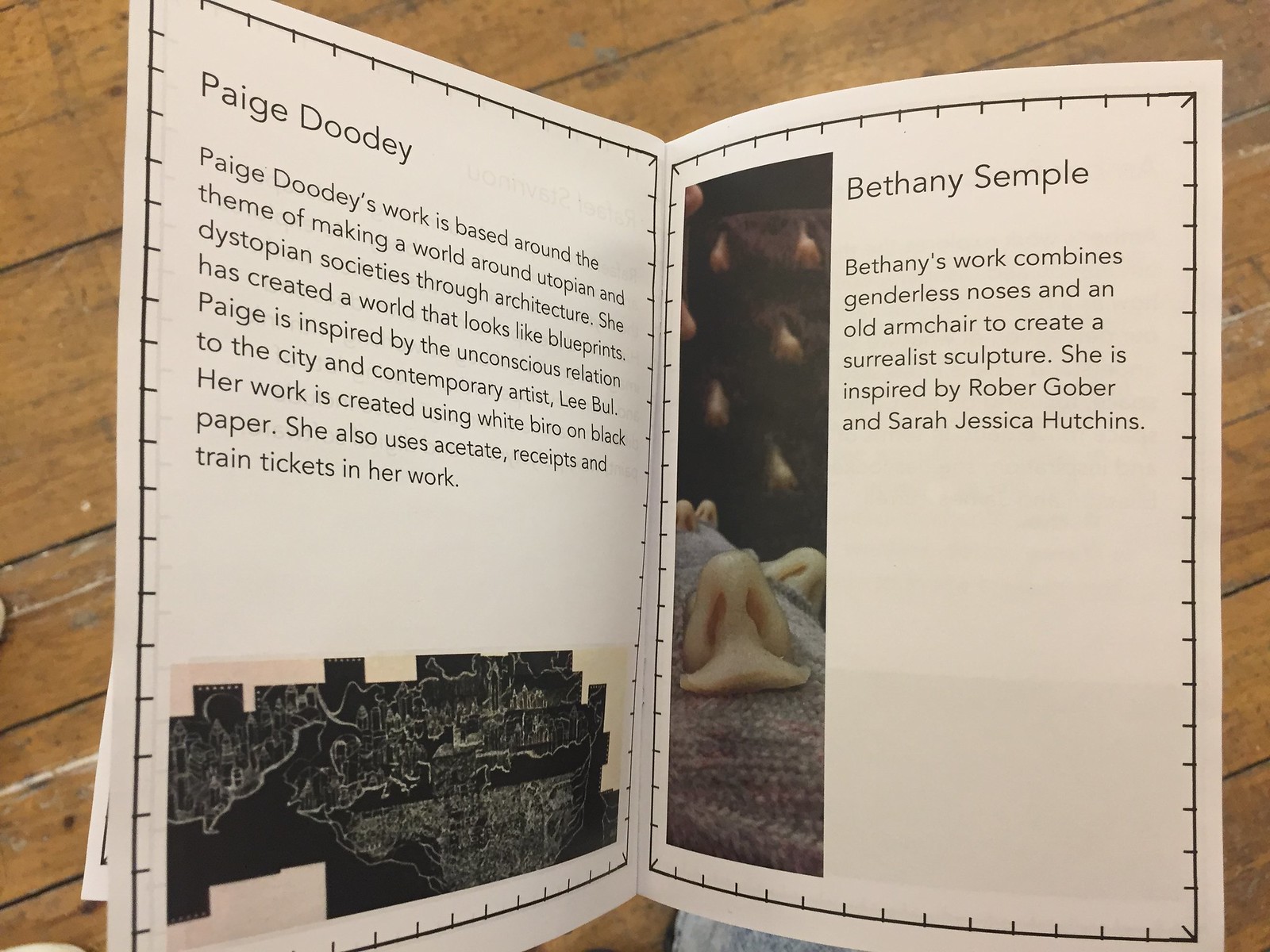The image features an open, handmade booklet with a white cover and black border design, placed on a wood surface, possibly the edge of a deck or table. The setup appears to be outdoors, likely during the daytime. The booklet, centered in the image, has two main pages displayed. On the left page, titled "Page Doody," the text describes Page Doody's work, which explores themes of utopian and dystopian societies through architecture, creating blueprint-like worlds. Her work utilizes materials such as white brio, black paper, acetate receipts, and train tickets, and is inspired by the unconscious relationship to the city and contemporary artist Lee Bull. The right page showcases Bethany Sample's work, which blends genderless noses and an old armchair into a surrealist sculpture, drawing inspiration from Robert Gober and Sarah Jessica Hutchings. The booklet's pages are adorned with a black outline, adding to its handcrafted feel. The surrounding colors in the image are predominantly brown, black, white, tan, and gray.